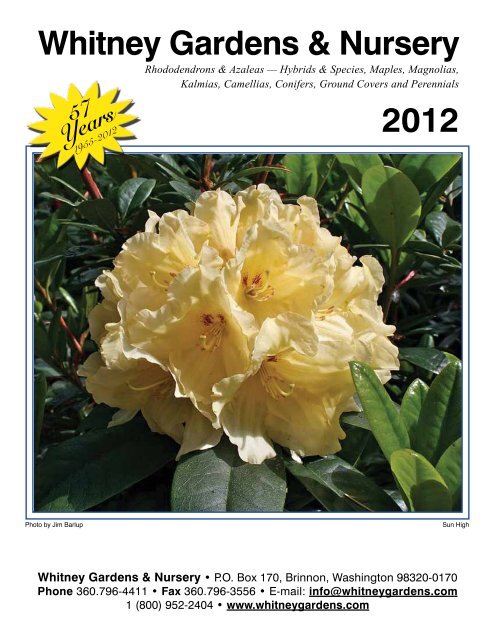The advertisement features a detailed layout for Whitney Gardens and Nursery. At the top, bold black letters read "Whitney Gardens and Nursery". Below that, in smaller black text are the words: "Rhododendrons and Azaleas, Hybrids and Species, Maples, Magnolias, Calmeas, Camellias, Conifers, Groundcovers, and Perennials". To the left, there is a yellow starburst with "57 years" in black lettering and the dates "1955-2012". On the right side, the year "2012" is printed in black. 

The centerpiece of the advertisement is a photograph depicting a cluster of white and possibly yellowish flowers with visible buds and stamens at their centers, surrounded by lush green foliage, giving an impression of a wild, natural setting. This floral arrangement appears like a circular bouquet with more flowers visible both above and below the primary cluster.

At the bottom of the ad, it reads "Whitney Gardens and Nursery, P.O. Box 170, Brinnon, Washington 98320-0170". Additional contact details are provided: phone number 360-796-4411, fax number 360-796-3556, email at info@whitneygardens.com, and a website, www.whitneygardens.com. On the bottom left of the image, the photo is credited to "Joe" whose last name is partially visible, and some small print appears on the bottom-right of the image as well.